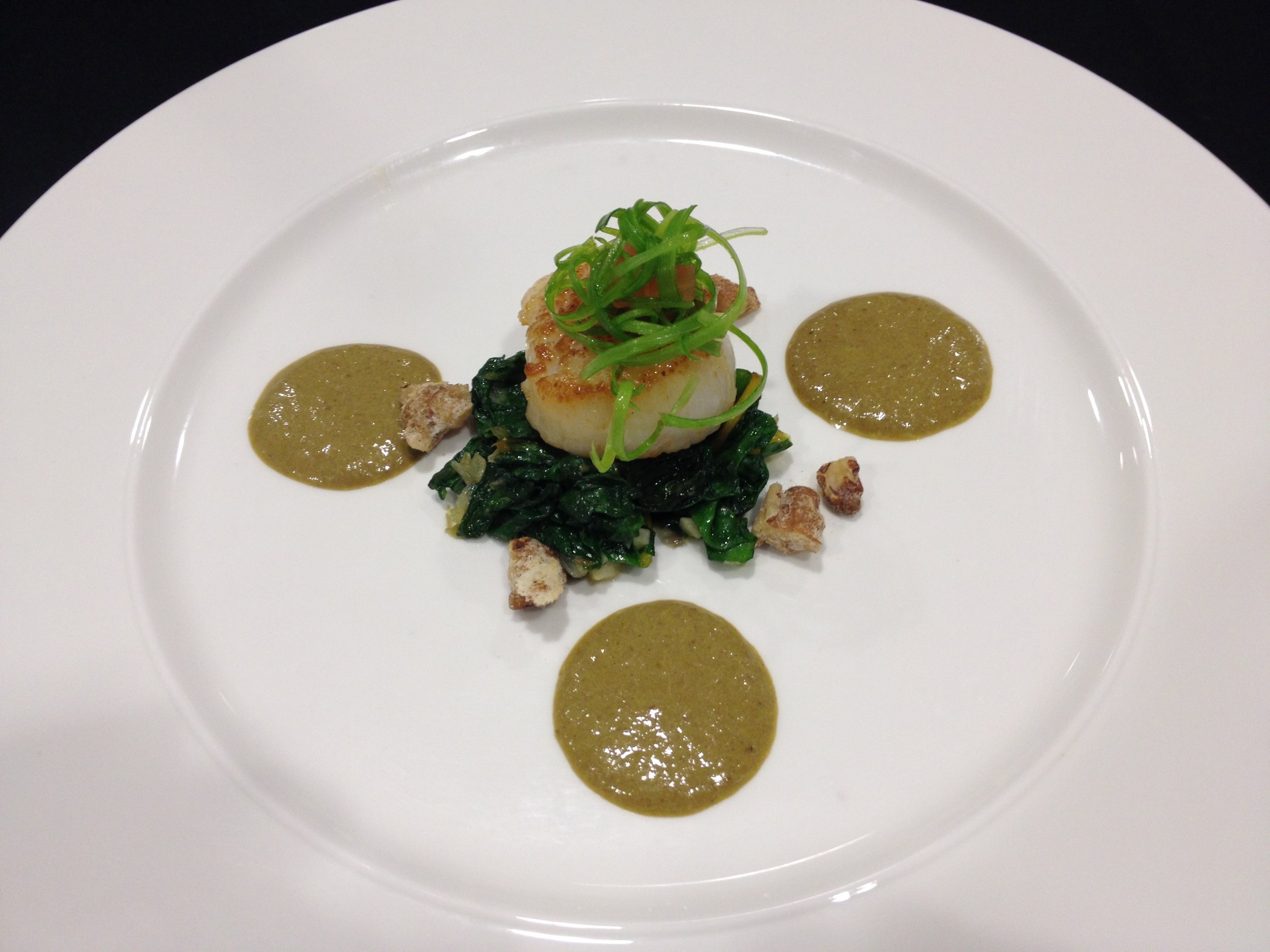This image is a color photograph of an exquisitely plated appetizer, centered on a pristine white plate that starkly contrasts with the black background, making the arrangement of the food stand out strikingly. Dominating the center is a perfectly seared scallop, featuring a golden-brown surface, resting on a bed of sautéed dark greens, likely seaweed or spinach. Delicately perched atop the scallop are finely shredded light green scallions, adding a touch of freshness and height to the presentation. Surrounding the scallop are four pieces of brown nuts, possibly walnuts, which add texture to the dish. Enhancing the visual appeal and flavor, there are three small, artistic dollops of a thick, green sauce that could be a variation of green goddess or a sophisticated vinaigrette. The sophisticated and minimalist presentation underscores its haute cuisine origins, making it clear that this elegant, bite-sized offering is designed as an appetizer, likely served at a Michelin-starred restaurant or for a gourmet menu photoshoot.